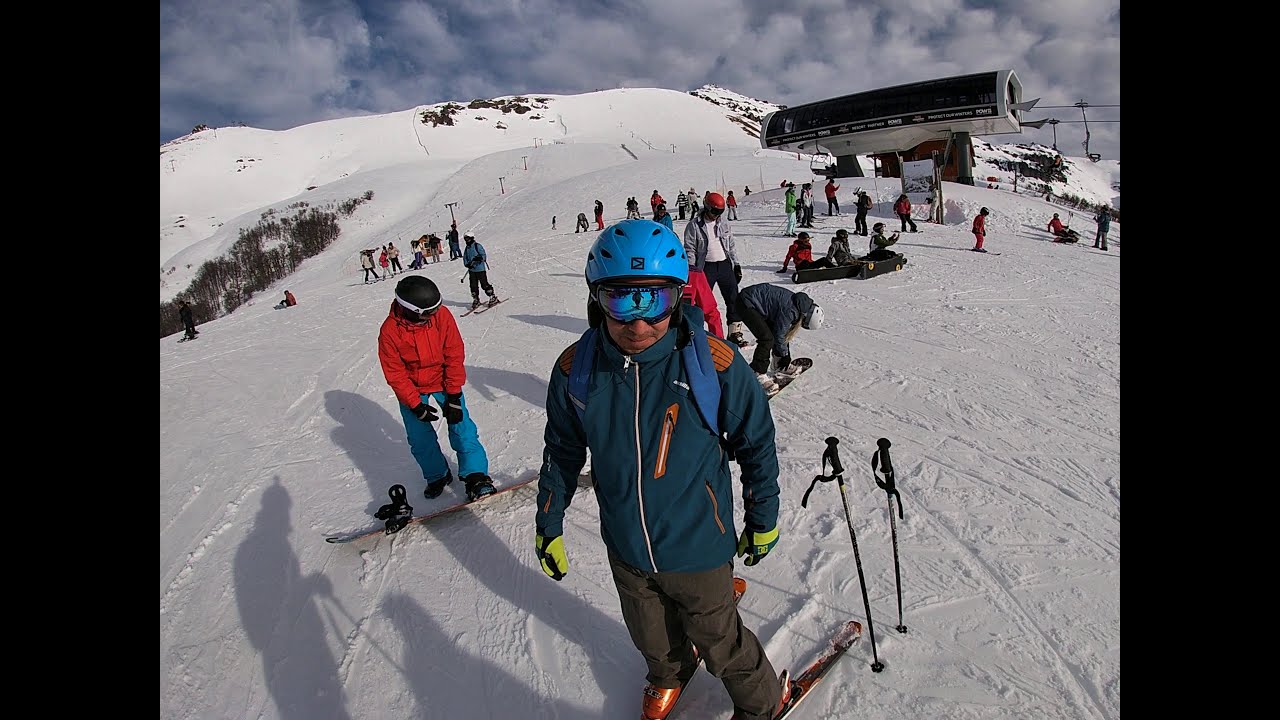The photograph captures a dynamic scene at the base of a snow-covered ski hill, bustling with activity. At the center foreground, a man stands prominently, facing the camera. He is outfitted in a blue jacket, gray ski pants, and a light blue helmet with coordinating blue goggles. His skis are affixed to his feet, and his poles are planted in the snow behind him. Surrounding him, a diverse group of about 20-25 people can be seen, either skiing down the hill or in various stages of preparing their snowboards and ski gear.

In the upper right of the image, there is a ski lift station with chairs extending out, likely ferrying skiers up the hill. Adjacent to it, there appears to be a covered structure, possibly a lodge or a sheltered resting area. Further up in the background, two snowmobiles are visible, suggesting the presence of ski patrol or maintenance staff.

The scene is set against a backdrop of a large mountain with a sky that is moderately cloudy, hinting at the high altitude. The photograph bursts with color, displaying outfits in shades of blue, red, black, neon yellowish-green, orange, and gray, all contrasting vividly against the white snow. The horizontal panoramic frame of the image captures the hustle and tranquility of this outdoor, daytime winter setting.